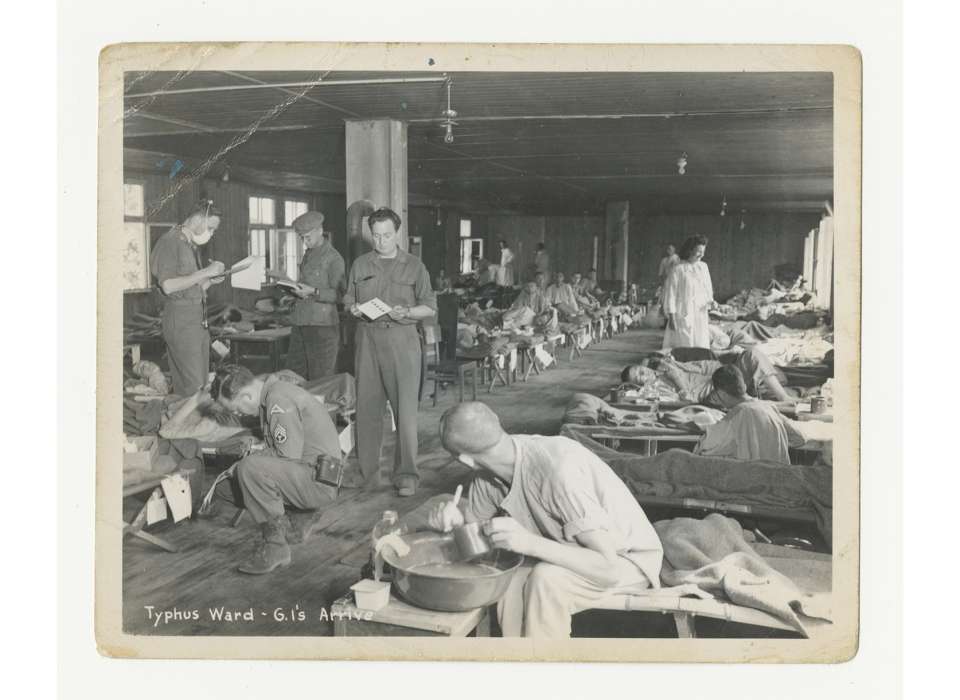This image is a black and white photograph, scanned and worn, depicting an old military hospital ward that appears to have been used for typhus treatment. Distinctive curls, rings, and creases mark the aged photo that rests on a white background. In the left-hand corner of the image, white text reads, "Typhus Ward - GIs Arrive," indicating the ward's purpose and the presence of military personnel.

The ward is vast and open, filled with narrow cots where sickly men, likely soldiers, are either lying down or sitting up. Many appear thin and are dressed in hospital garments. In the foreground, one man is drinking or washing from a small metal bowl. In the distant background, some figures in white, presumably nurses, are walking between the cots, attending to the patients.

A prominent support pole is visible, and near it, a couple of military men are kneeling, wearing uniforms with visible rank patches, reading and possibly assisting with medical duties. The scene captures a moment in which soldiers afflicted by typhus are being tended to in an organized, albeit crowded, medical environment.